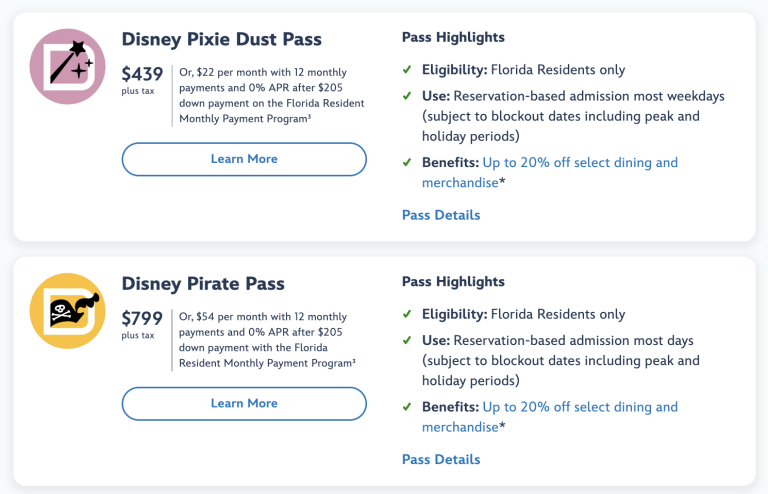The image consists of two sections highlighting different Disney annual passes. 

The top section presents information about the "Disney Pixie Dust Pass." It includes black text with some blue highlights and a white "Learn More" button featuring blue text. The pass is priced at $439 plus tax, or it can be financed at $22 per month with 12 monthly payments and zero APR after a $205 down payment, through the Florida Resident Monthly Payment Program. An icon with a "D" inside a purplish-pinkish circle is also present. The "Pass Highlights" specify that the eligibility is restricted to Florida residents only, and the use is reservation-based admission on most weekdays, subject to blackout dates including peak and holiday periods. The benefits include up to 20% off select dining and merchandise.

The bottom section describes the "Disney Pirate Pass." This pass costs $799 or can be financed at $54 per month with 12 monthly payments and zero APR after a $205 down payment through the same payment plan. The "Pass Highlights" for this option also state that eligibility is restricted to Florida residents only, and use is reservation-based admission on most days, subject to blackout dates including peak and holiday periods. Benefits are similarly up to 20% off select dining and merchandise. There is another white "Learn More" button with blue text, and a "Pass Details" section available for more information.